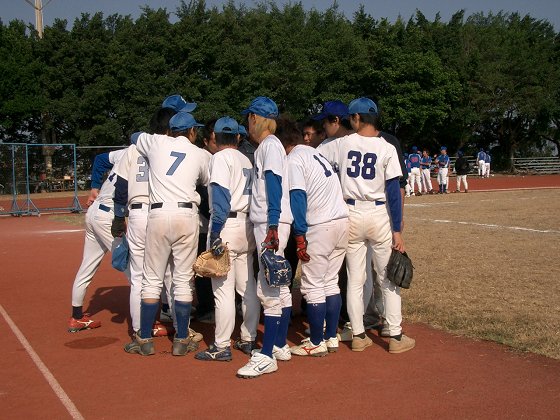The photograph captures a group of baseball players huddled together with their backs facing the camera, forming a circular arrangement. They are outfitted in coordinated white uniforms, consisting of short-sleeved t-shirts with visible numbers on the back – notably 3, 7, 11, and 38 – under which some wear long-sleeved blue shirts. Their white pants are complemented by belts and knee-high blue socks, and footwear varies from brown, white, to red shoes. Blue baseball caps cover their heads, and a few players can be seen holding baseball gloves. The scene is set outdoors on a baseball field that features patches of both yellow and green natural grass, intersected by white painted lines. This field is encircled by a tan hard surface track marked with white lines. In the far background, a dense treeline with lush green foliage is visible under a light blue, cloudless sky. Additional activity is discernible in the upper right quadrant of the image, indicating the presence of another team.